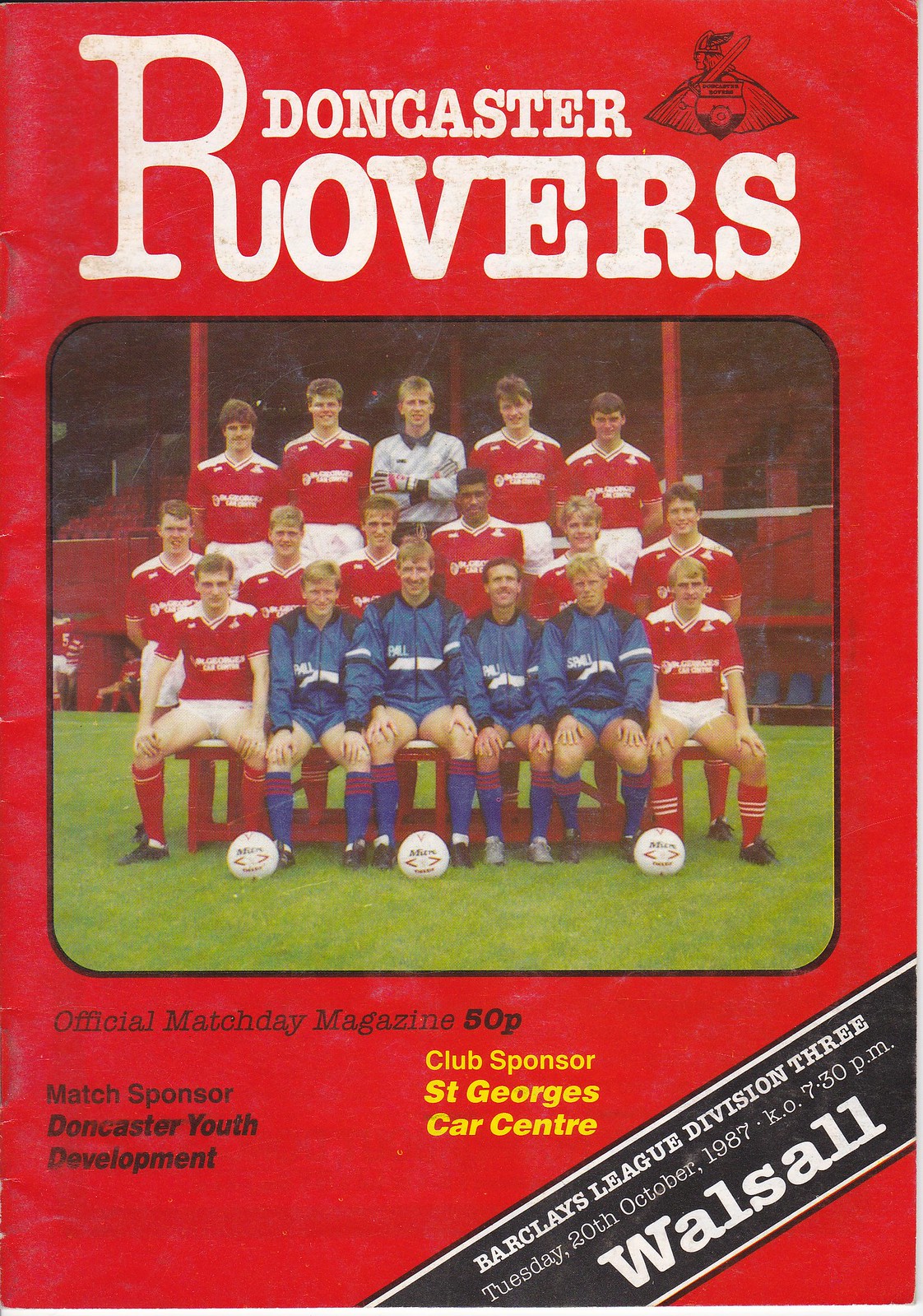The front cover of this vintage sports magazine features a red, slightly creased background with "Doncaster Rovers" prominently displayed at the top in giant white letters. To the top right, the Doncaster Rovers' black logo, resembling a Viking with a shield, faces left.

At the center of the cover, a rounded-corner square image with a black border depicts a soccer team posing for a photo. The photograph showcases a diverse team, primarily clad in red and white jerseys, standing in three rows. In the front row, four men are seated on a red bench, distinctively dressed in long blue jackets, blue socks, and shorts, contrasted by two men at the edges wearing the standard red team uniform. Three white soccer balls rest on the vividly green grass in front of them. The second and third rows consist entirely of men in the traditional red and white uniform, except for one individual in the center of the third row wearing a white shirt with black details.

Beneath the photograph, black text declares, "Official Match Day Magazine 50p, Match Sponsor Doncaster Youth Development," followed by, "Club Sponsor St. George Car Center" in yellow. A black bar spans the bottom of the cover, adding a finishing touch to this nostalgic sports memorabilia.